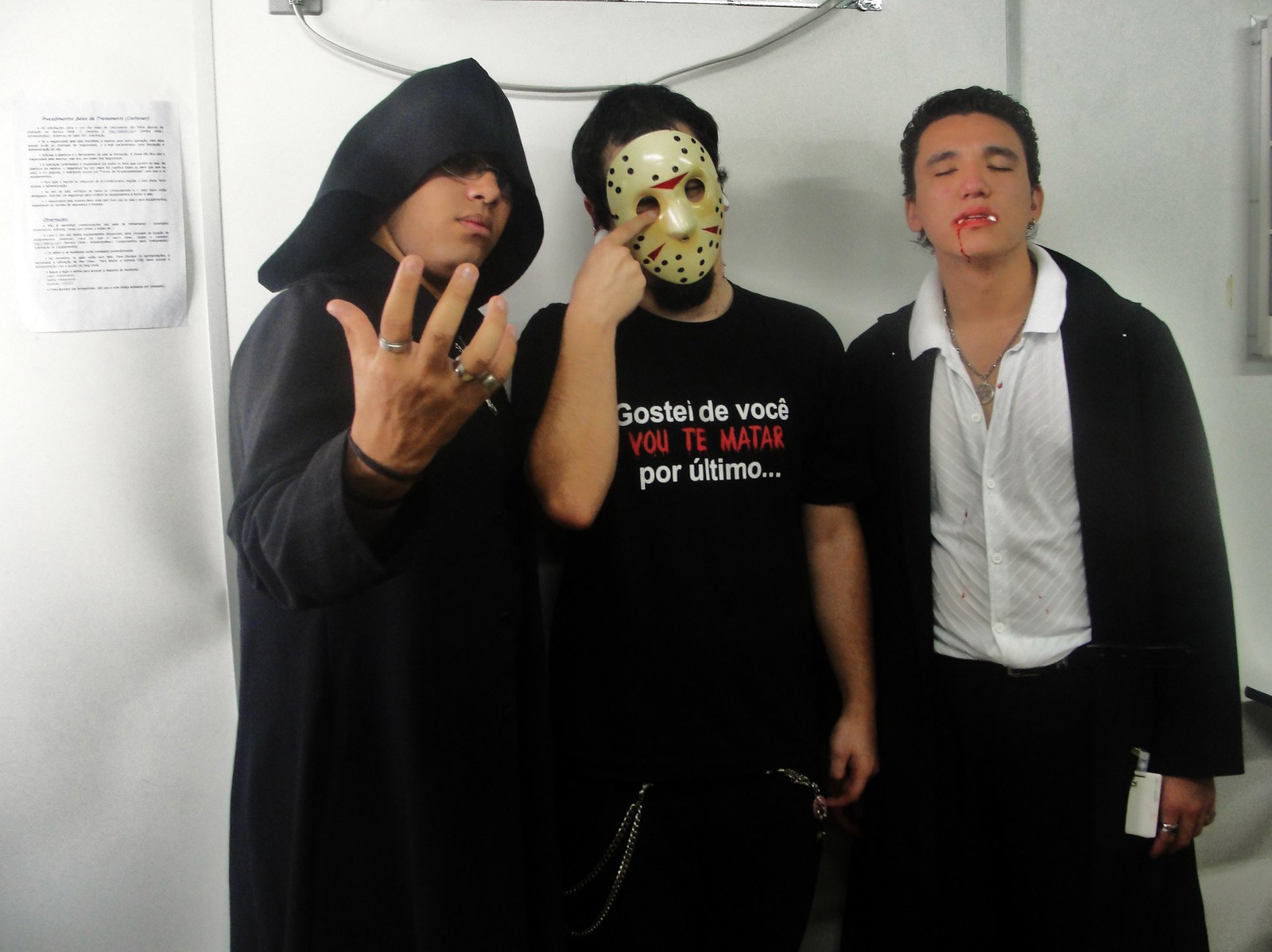This detailed photograph depicts three young adult males dressed in Halloween costumes, captured in what appears to be a workplace setting, evident by the presence of an ID badge and an official-looking memo on the wall behind them. The young man on the left is clad in a long black tunic reminiscent of a Grim Reaper, with a hood casting shadows over his eyes. He has his right hand raised, adorned with silver rings on three fingers, giving him an ominous appearance. The man in the center dons a hockey mask resembling Jason Voorhees from Friday the 13th, holding it up with one finger pointing at his right eye. He wears a black t-shirt with white and red writing in an unfamiliar language ('Gosta de voce voce matar por ultimo') and black pants accessorized with chains. The third gentleman on the right portrays a vampire, evident by his fake fangs and faux blood dripping from the corner of his mouth. He wears a black jacket over a white shirt. Despite the Halloween-like costumes, the photo might depict another type of celebration, possibly outside the United States, suggested by the foreign language text on the central figure's shirt.